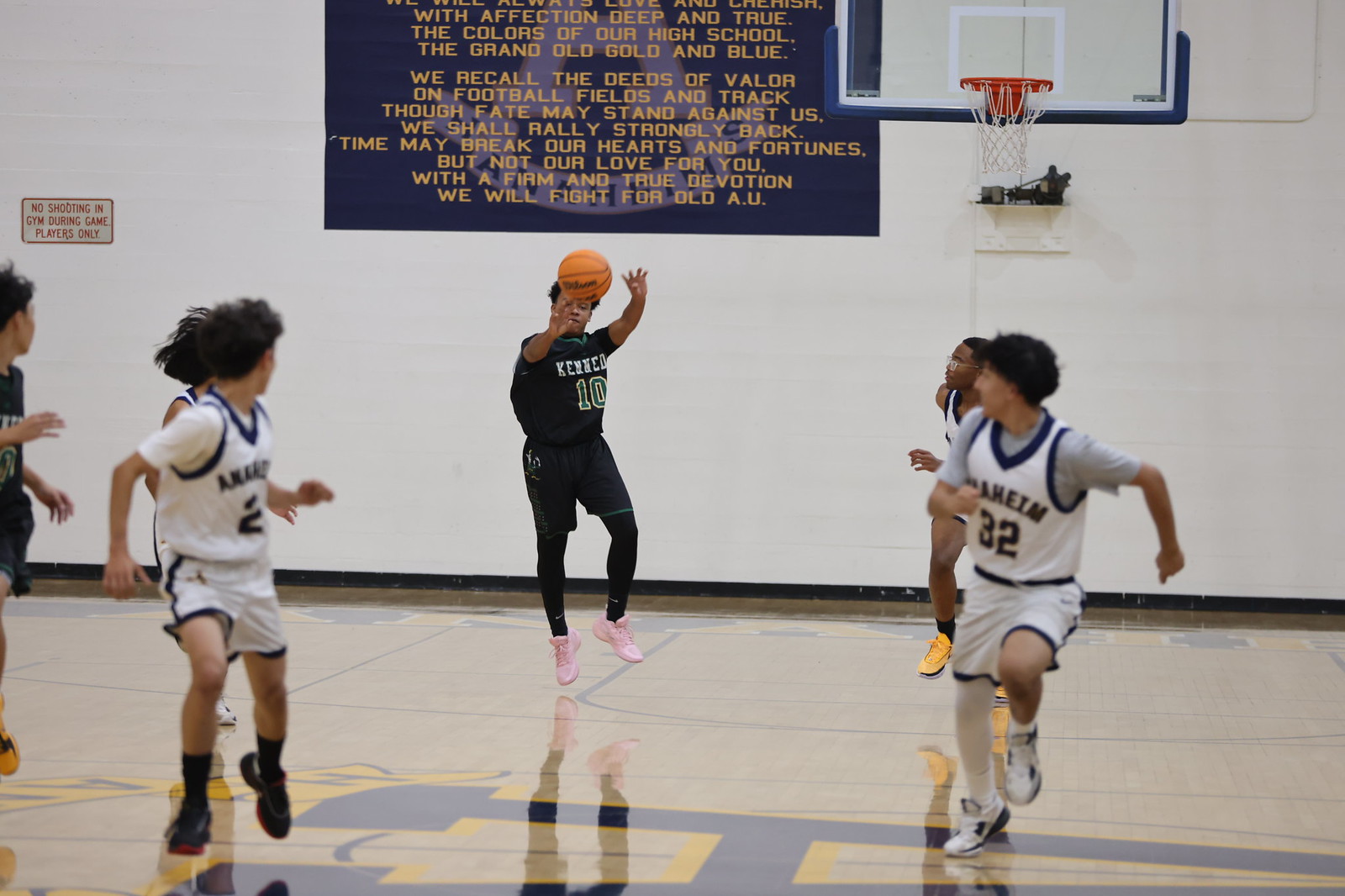The photograph captures an intense moment during a high school basketball game. In the scene, one team is dressed in black jerseys accented with a hint of green, while their opponents don predominantly white jerseys with blue accents. Central to the image is a player from the black team preparing to pass the ball to a teammate positioned near midcourt, yet still within the backcourt area. 

The players from the white team appear to be strategically positioned, with four of them dispersed but collectively focused towards the central area of the court. An 'A' is prominently displayed on the floor at midcourt, possibly indicating the school's initials. 

In the background, there is a banner hanging on the wall, likely showcasing school pride or information about the game. The angle of the photograph also provides a clear view of one of the basketball hoops, further grounding the viewer in the setting of the gymnasium. This detailed scene encapsulates the dynamic and competitive nature of high school basketball.